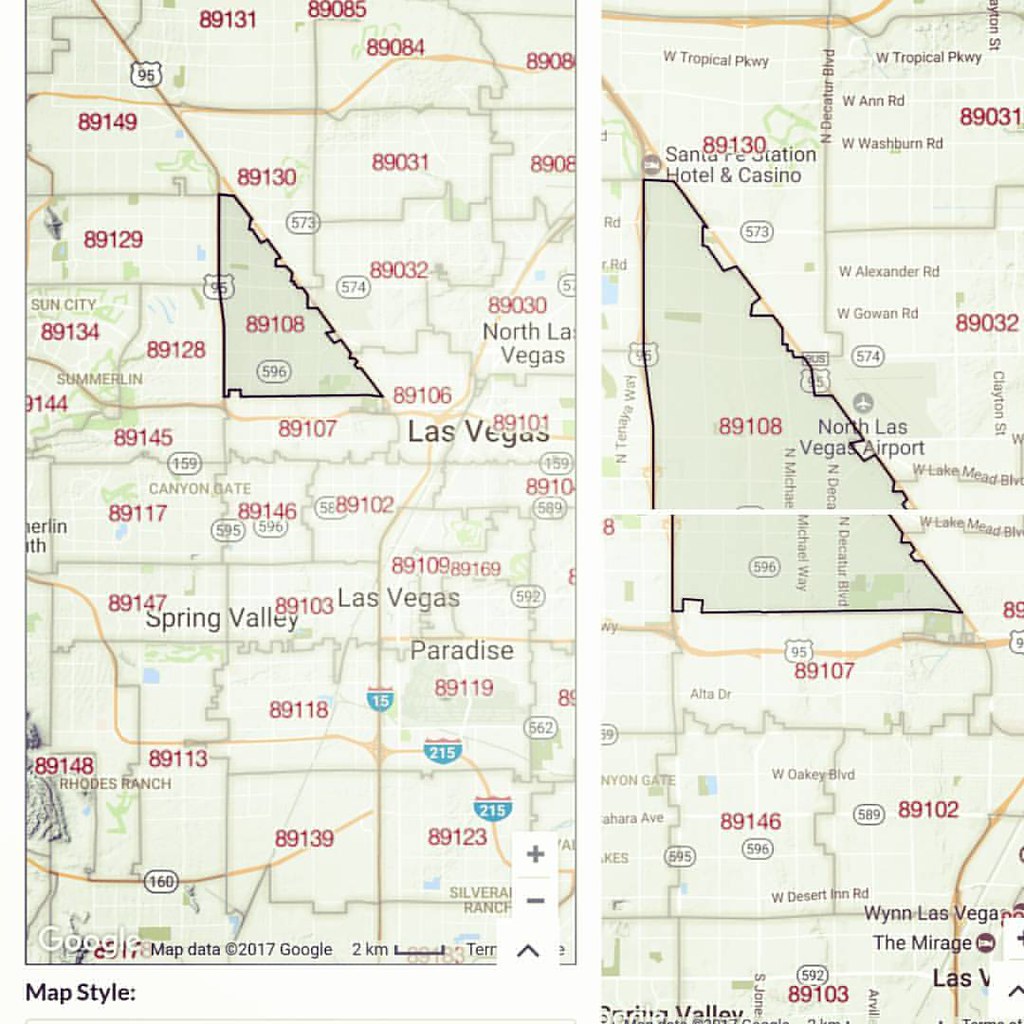This color image, presented in a square format, appears as a composite of three related segments. The largest section on the left features a computer-generated map of Las Vegas. This overview map displays various neighborhoods, each separated by distinct five-digit ZIP codes such as 89108 and 89107 but lacks intricate details.

To the right, a narrower segment showcases an enlarged view of one specific neighborhood, the 89108 ZIP code, providing a more detailed look at this area. Notably, the North Las Vegas Airport is visible in this zoomed-in section, a feature not discernible in the broader map due to the scale.

Beneath this is another connected image, acting as a continuation of the detailed section. It further explores the 89108 neighborhood, offering additional cartographic detail that could not be encapsulated within the bounds of the single zoomed-in segment. Collectively, these images provide a layered visual representation of Las Vegas, from a broad overview to finely detailed neighborhood specifics.